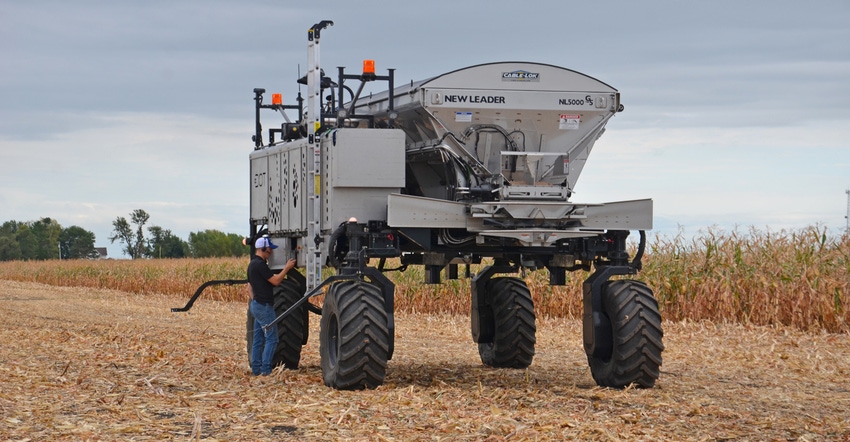The image is a color photograph depicting a large farming tractor in an expansive cornfield under a light blue-gray sky with scattered white clouds. The scene is detailed with green trees and bushes on the left, and a ground cover on the right that appears to be a combination of fallen leaves or corn husks, with a visible field of corn stalks that are green but turning brown at the base. The tractor is a towering farm machine, at least 10-12 feet high, equipped with four large, aggressive rubber tires that elevate it off the ground. Prominently displayed on the tractor's front is the text "New Leader NL 5000" in black. The vehicle, constructed of heavy-duty steel, has a side ladder and is being operated by a man clad in dark blue jeans, a black shirt, and a white hat, who appears to be pressing buttons on the side. The expansive background reveals an unharvested cornfield stretching over numerous acres, framed under a daylight sky tinged with light clouds.